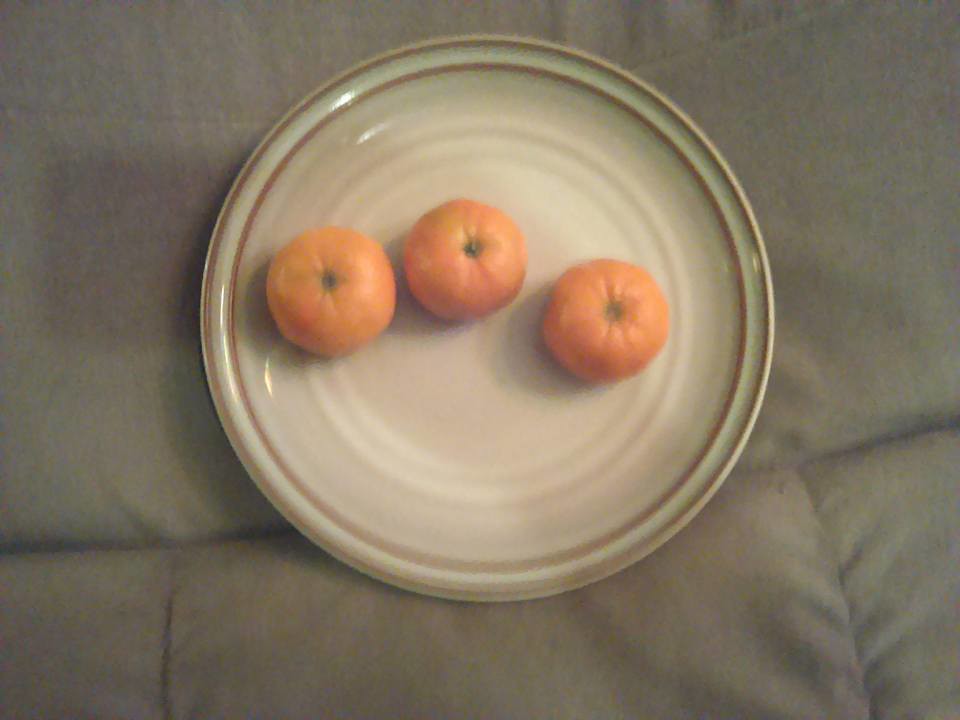This extreme close-up photograph, slightly out of focus but clear enough, presents a bird's eye view in landscape format. The scene captures a thick, white bedspread adorned with visible folds and creases, suggesting the surface is a bed—possibly a duvet or bed topper. Atop this bedspread rests a ceramic plate, predominantly white with detailing consisting of two brownish rings: one circling the edge and the other slightly inward. Displaying a handmade aesthetic, this sturdy plate holds three bright orange clementines, each with evident stem indentations but unpeeled and pristine.